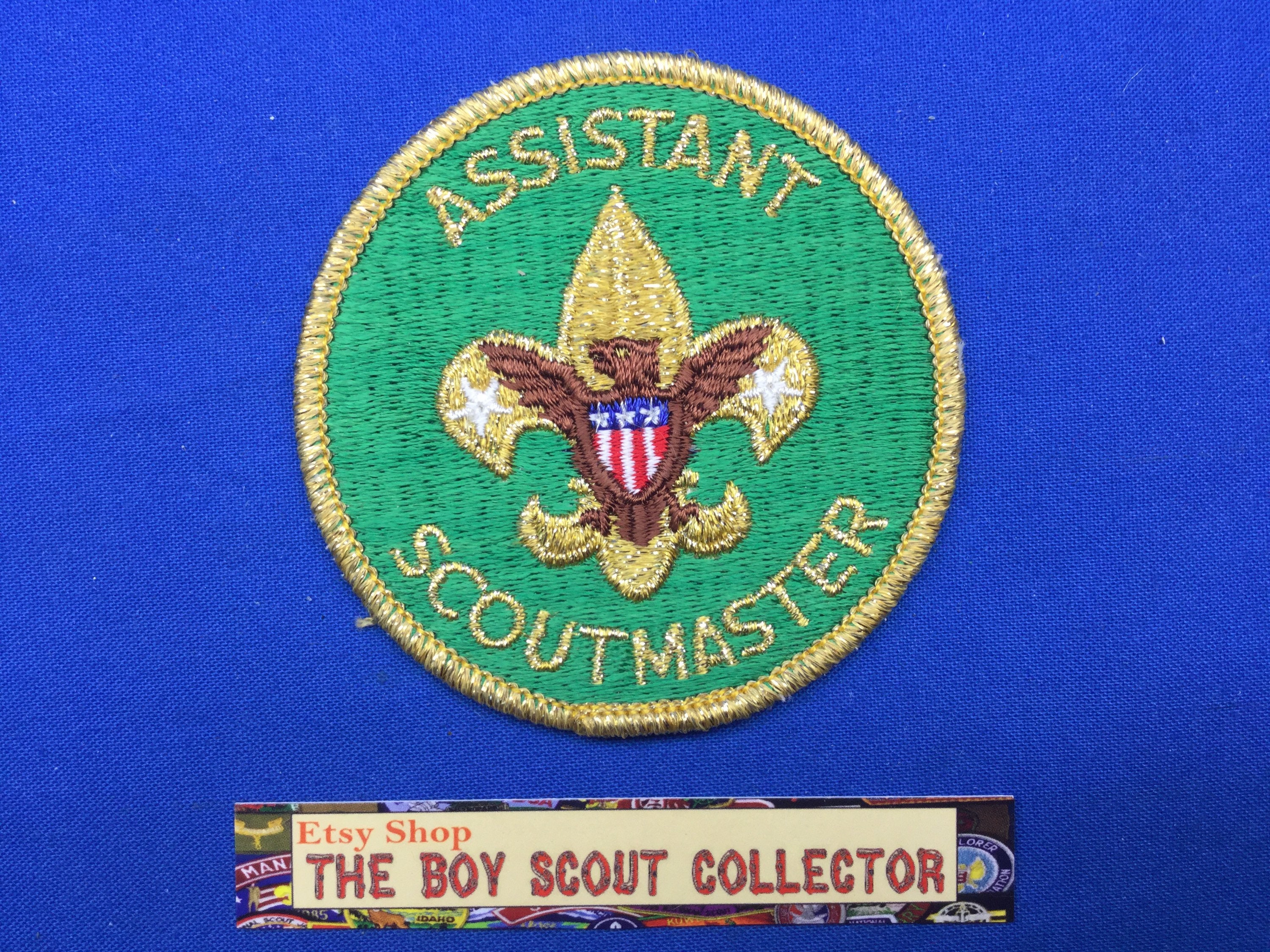This image features a detailed, round embroidered patch intended for an Assistant Scoutmaster. The patch itself has a light green base with a gold border. Prominently displayed in gold text, the words "Assistant Scoutmaster" encircle the center, where a large gold fleur-de-lis is situated. Embedded within the fleur-de-lis is a brown eagle facing left, which bears a shield on its chest. The shield is detailed with three white stars on a blue field at the top, and red and white stripes below. Beneath the patch is a label that reads "Etsy Shop: the Boy Scout Collector" in orange and red text on a white banner-like background, all set against a royal blue fabric backdrop.